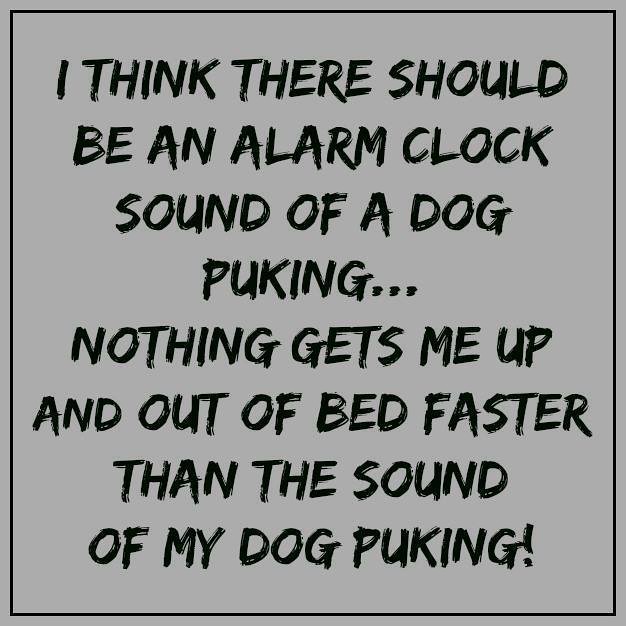The image features a humorous, computer-generated digital message on a gray background. It is framed by a thin black border. The text, displayed in all capital letters, reads: "I THINK THERE SHOULD BE AN ALARM CLOCK SOUND OF A DOG PUCKING. NOTHING GETS ME UP AND OUT OF BED FASTER THAN THE SOUND OF MY DOG PUCKING!" The text appears in a rugged, paintbrush-like font, with parts of the letters appearing lighter, as if the "paint" didn't fully adhere. This meme-style image is crafted for sharing on social media platforms like Facebook and Instagram, aiming to elicit laughs through the relatable panic induced by the sound of a dog about to vomit.